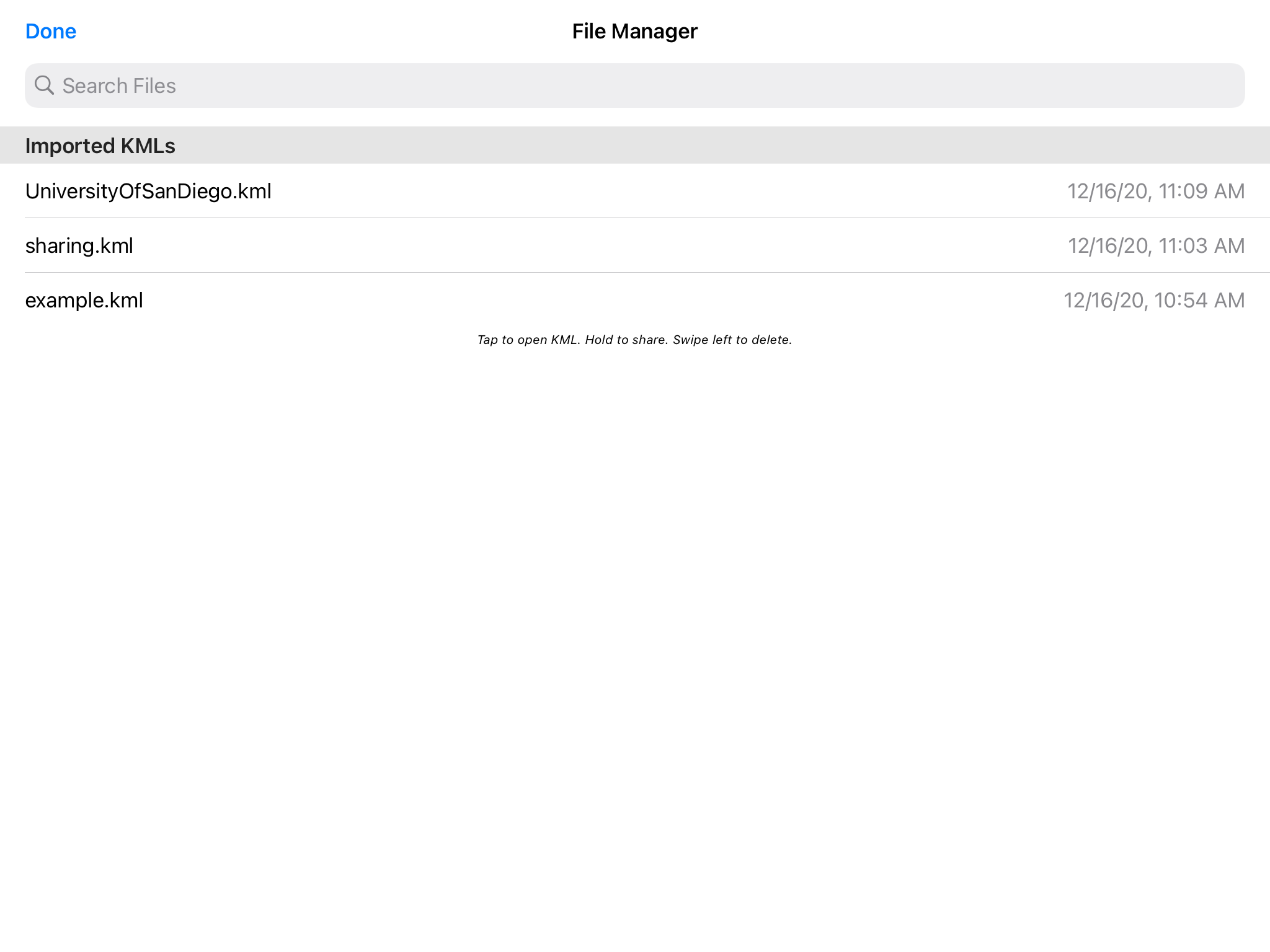The image is a cropped screenshot showcasing the file manager interface for KML (Keyhole Markup Language) files, commonly used with Google Earth. In the top left corner of the screen, a bold, light blue "Done" button is prominently displayed. Centered at the top, the title "File Manager" is written in bold black font. Directly below the title is a large search bar with the placeholder text "Search files."

Beneath the search bar, there is a prominent gray banner that reads “Imported KMLs” in the top left corner. Following this banner is a vertical list of imported KML files. The first file listed is "universityofsandiego.kml," which was imported on December 16, 2020, at 11:09 AM. The second file, "sharing.kml," has an import timestamp of 11:03 AM on the same date. The third and final entry is "example.kml," imported on December 16, 2020, at 10:54 AM. Each file entry includes its respective import date and time on the right side of the interface.